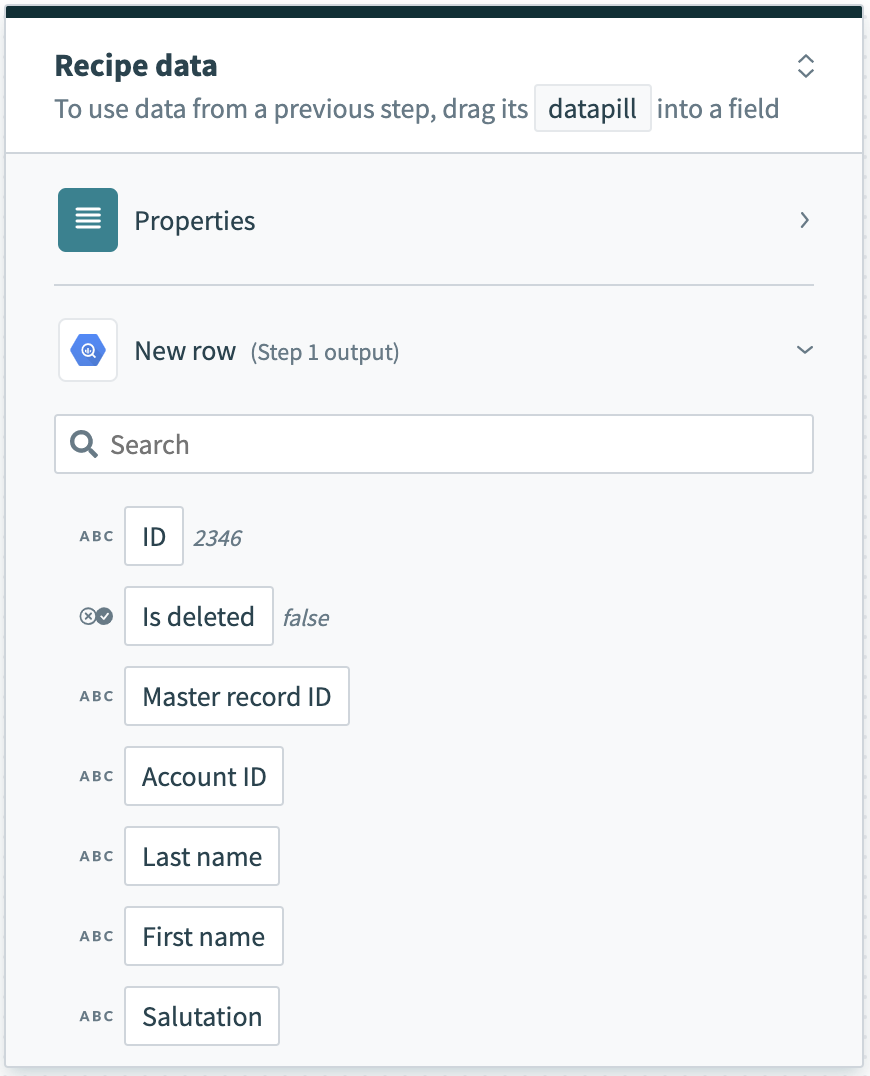The image displays a white square form with a structured layout predominantly featuring text and buttons. At the top, it is headed by the title "Recipe Data" in bold black font. 

Below the title, an instructional sentence reads: "To use data from a previous step, drag its data pill into a field," with "data pill" specifically highlighted in bold black text, while the rest of the text is in light gray.

Beneath this instruction, there is a prominent dark green square button with white stripes across its center, labeled "Properties." Adjacent to this, a white square button features a hexagonal icon containing a microscope image. This button is labeled "New Row (Step 1 Output)."

Further down, a search bar is discernible, consisting of an icon of a magnifying glass next to the word "Search."

The following interface elements are arranged in a column:

1. A button labeled "ABC."
2. A square with "ID" written inside, followed by the number sequence "2346."
3. An icon showing a circled X and a circled check mark next to a rectangle labeled "Is Deleted," with text indicating "False" next to it.
4. "ABC" in small capital letters, followed by a rectangle labeled "Master Record ID."
5. Another "ABC" in small capital letters, followed by a rectangle labeled "Account ID."
6. Again, "ABC" in small capital letters, followed by a rectangle labeled "Last Name."
7. "ABC" in small capital letters, followed by a rectangle labeled "First Name."
8. Lastly, "ABC" in small capital letters, followed by a rectangle labeled "Salutation."

This comprehensive layout forms the bottom of the visual content.